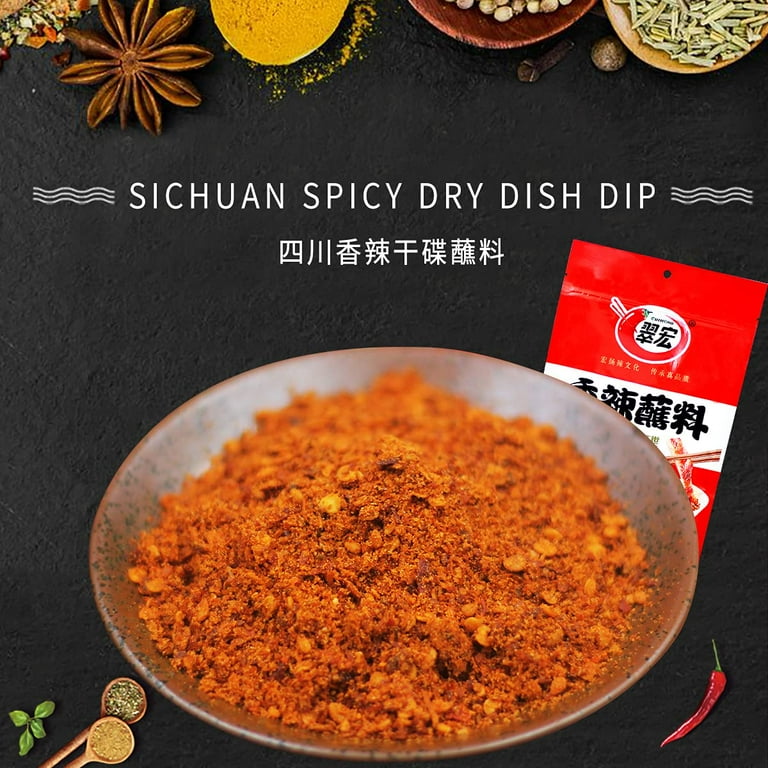This image appears to be an advertisement, potentially even the packaging, for a product titled "Sichuan Spicy Dry Dish Dip" with the same title repeated in Chinese characters. The background is predominantly black, enhancing the contrast and visibility of the vibrant elements in the foreground. The focal point is a large ceramic bowl, placed in the center, heaped with an orange, chunky, and richly textured spice blend, indicating its spicy nature. The packaging of the product, which is red and white with Asian letters, is partially visible behind the bowl.

Above the bowl, the illustration showcases an array of natural ingredients that are likely components of the dip. These include vivid depictions of chili peppers, star anise, cloves, fennel, coriander seeds, and turmeric, which are meticulously arranged to underline the freshness and exotic appeal of the spices. Tucked in the bottom right corner of the image is a red chili pepper, while the bottom left corner features two teaspoon measuring spoons—one with a green-colored spice and the other with a yellow spice—alongside some leafy herbs, possibly basil. This detailed arrangement, accentuating a diverse palette of flavors and colors, emphasizes the authenticity and spiciness of the Sichuan Spicy Dry Dish Dip, making it look both enticing and vividly flavorful.